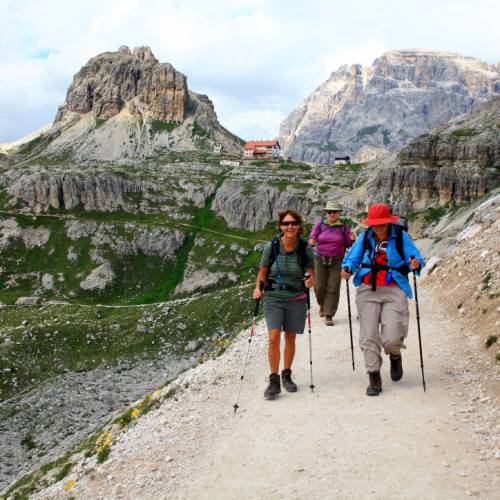In this vibrant daytime image, three middle-aged women are captured trekking on a rugged mountain trail, sharing a moment of laughter and camaraderie as they walk towards the camera. The woman at the back wears a purple shirt and brown pants, while the woman on the left sports a green shirt with matching shorts, high boots, and uses walking sticks. The woman on the right is clad in a blue jacket over a red shirt, paired with gray pants. The trail they traverse is surrounded by rocky terrain interspersed with patches of green grass. The backdrop features a series of majestic mountains and three isolated buildings, including one with a red roof that resembles a large house or possibly a touristy hotel, adding a curious element to the serene landscape.